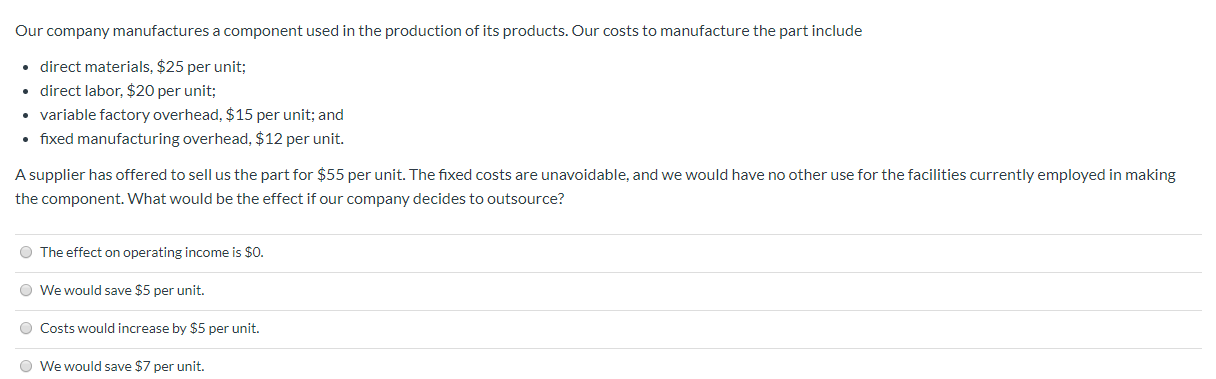This photograph captures a multiple-choice question presented in text form on a white background with small black fonts. The text outlines a scenario where a company manufactures a component for its products. The detailed cost breakdown for manufacturing the part includes direct materials at $25 per unit, direct labor at $50 per unit, variable factory overhead at $15 per unit, and fixed manufacturing overhead at $12 per unit. An external supplier has offered to sell the part for $55 per unit. It is noted that the fixed manufacturing costs are unavoidable, and there is no alternative use for the facilities currently used for production. 

The question posed is: "What would be the effect if our company decides to outsource?" Beneath this, four vertically arranged answer choices are available, each with a gray circle to its left for selection. The possible answers are: 

1. The effect on operating income is zero.
2. We would save $5 per unit.
3. Costs would increase by $5 per unit.
4. We would save $7 per unit. 

This clear and concise layout is designed for easy selection, making it straightforward to identify the best response based on the given cost analysis.